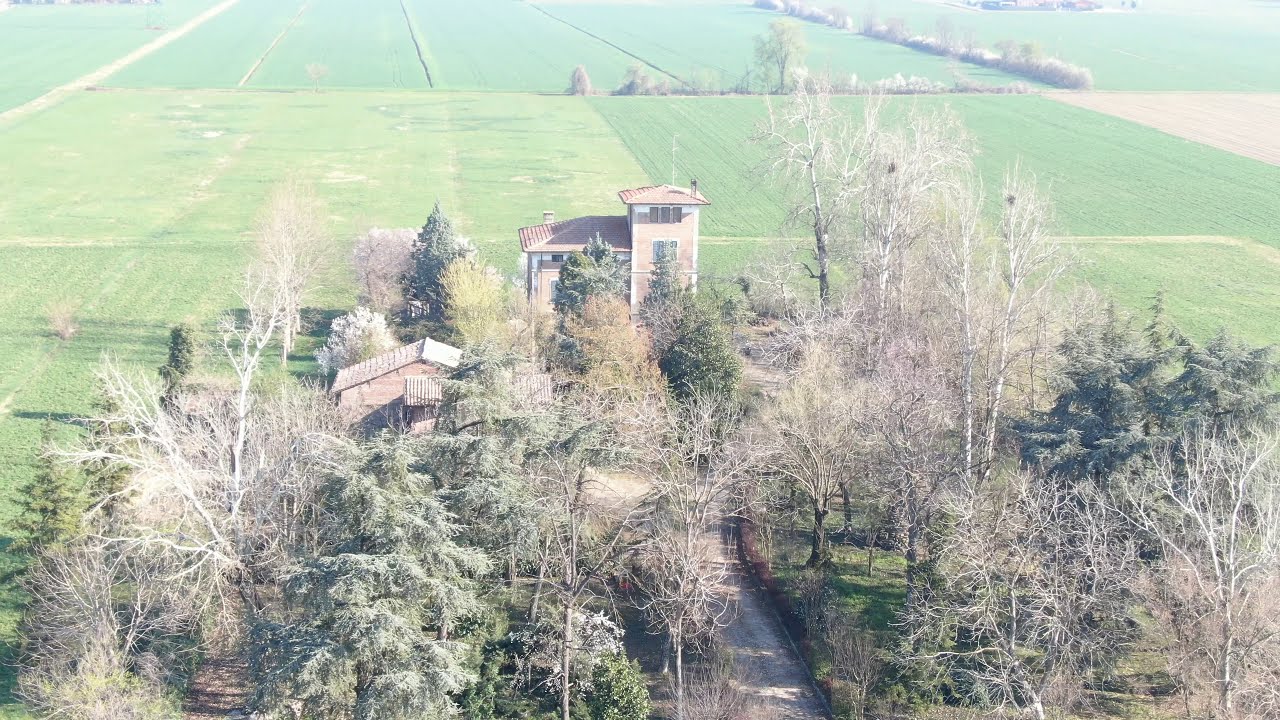The image depicts a large, two-story house with a tan exterior and tiled roofing, set in a sprawling landscape filled with greenery on a bright, sunny day. The house features a distinct square column on the side that extends an additional story above the main structure, making it three stories high. The driveway, made of dirt, winds up to the house and is flanked by multiple trees, some of which obscure parts of the house and driveway. Surrounding the house are several vast green fields, sectioned off and appearing to have been recently tilled by a tractor, ready for planting. To the right of the driveway, a sizeable grassy area interspersed with more trees can be seen. Behind the house and extending into the distance are numerous clusters of trees and extensive acres of mowed grass. A detached garage sits about 200 feet from the house, connected by a walkway through the trees. The image also captures a one-lane dirt road running alongside the left side of the property, further enhancing the rural and serene atmosphere of the scene.